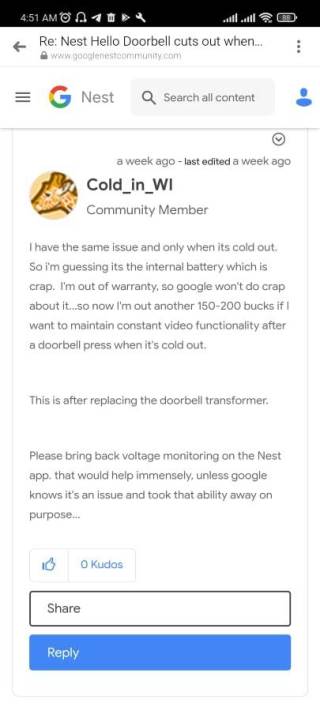This is a vertically oriented, rectangular cell phone screenshot. At the top, a black horizontal bar displays the time, 4:51 AM, along with the battery indicator on the right, and various small icons spread throughout. Below this bar, a light gray arrow points left next to the text “RE," followed by "Nest Hello Doorbell cuts out when" without any completion.

Directly beneath, the iconic multi-colored Google 'G' logo appears next to the word "Nest," adjacent to a search bar labeled "search all content." On the right side of the search bar, there is a blue or light blue icon resembling a person.

Under the search bar, the text reads, “a week ago, last edited a week ago.” Below this, a small circle appears, followed by a line of text that seems to depict an animal and the username “cold_in_WI_community_member” in black font.

The next segment in gray or black font reads, "I have the same issue and only when it's cold out. I'm guessing it's the internal battery, which is crap. I'm out of warranty, so Google won't do crap about it. Now, I'm out another 150 to 200 bucks if I want to maintain constant video functionality after a doorbell press when it's cold out. This is after replacing the doorbell transformer. Please bring back the voltage monitoring on the Nest app. That would help immediately unless Google knows it's an issue and took that ability away on purpose.”

At the bottom of the screenshot, options to “share” or “reply” are available.